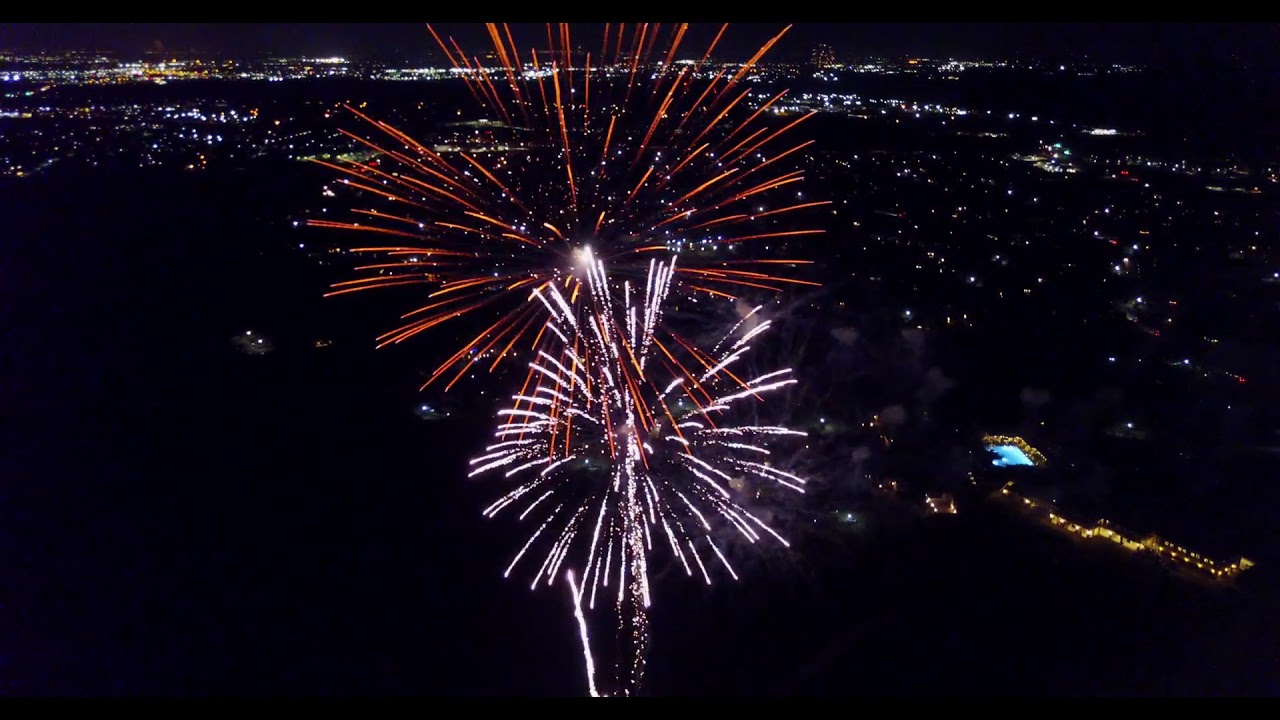Captured from a high vantage point, possibly by a drone, this landscape-oriented nighttime photograph showcases a sprawling cityscape awash with countless twinkling lights from buildings, streets, and residential areas. The centerpiece of the image is a stunning display of fireworks, with orange and white explosions prominently lighting up the sky. Smaller pink and white bursts can be seen in the foreground, adding depth and contrast. Near the bottom and to the right, a small, illuminated swimming pool colored in a distinctive bluish hue stands out amidst the sea of lights. The top left of the image transitions into a denser cluster of city lights, hinting at more urban structures, while the bottom left fades into near-complete darkness. This photograph encapsulates the breathtaking spectacle of a city alive with lights and celebrations, set against the still canvas of the night.